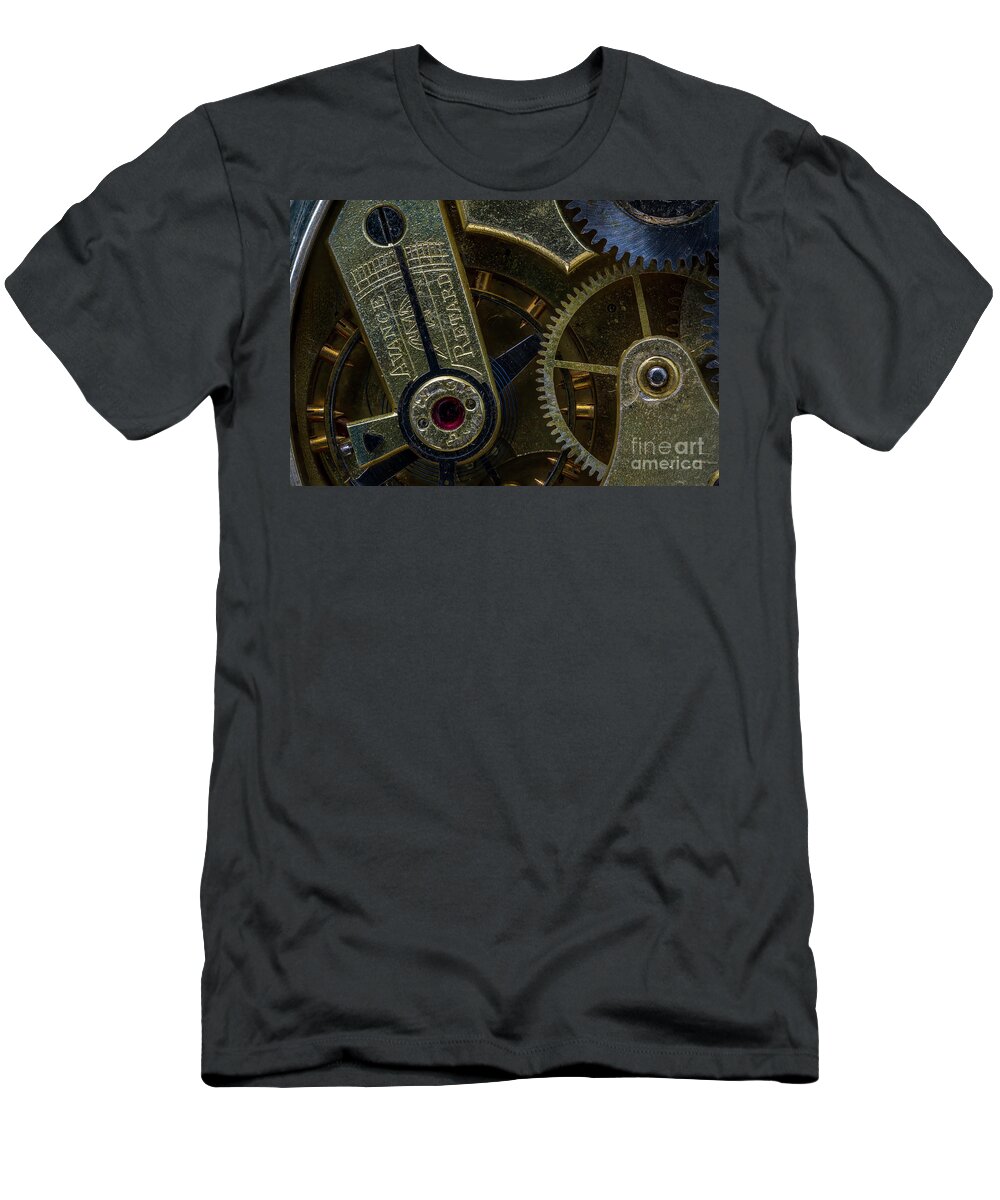The photograph features a dark grey, short-sleeved t-shirt with a crew neck, lying slightly wrinkled on a featureless white background. The t-shirt's chest is adorned with a rectangular photographic image depicting intricate clockwork machinery. This detailed graphic includes various gears and a flywheel, primarily in shades of light and dark grey, with notable elements like a blue cog. Additionally, there are hints of bronze, gold, and even a touch of red within the machinery. Some text inscribed on the machinery reads "A-V-A-N-C-E retard." The lower right corner of the image prominently displays the logo for Fine Art America.